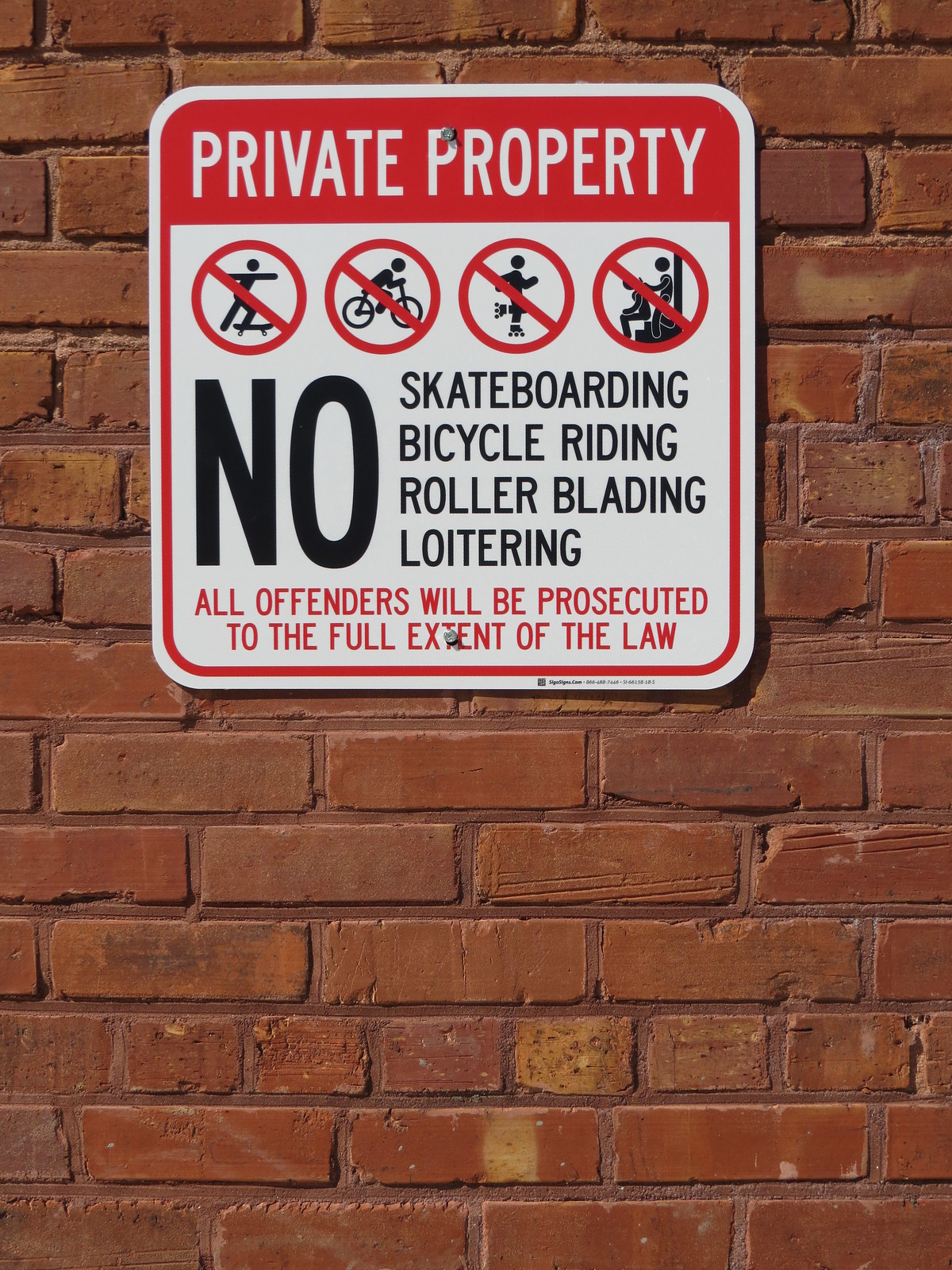This photograph captures a common warning sign bolted into a brick wall, positioned in the upper half of the image. The metal sign prominently features the words "PRIVATE PROPERTY" in white capital letters on a red stripe, which is framed by a red border around the white body of the sign. Directly below this header, there is a clear international no symbol—a red circle with a diagonal line—encompassing four black stick figure icons: one skateboarding, one riding a bicycle, one rollerblading, and one loitering. Adjacent to these icons, the sign clearly states in bold black letters: "No Skateboarding, Bicycle Riding, Rollerblading, Loitering." Beneath this, in red lettering, the sign warns: "ALL OFFENDERS WILL BE PROSECUTED TO THE FULL EXTENT OF THE LAW." The sign is secured to the wall with metal screws, making its prohibitions unmistakable.